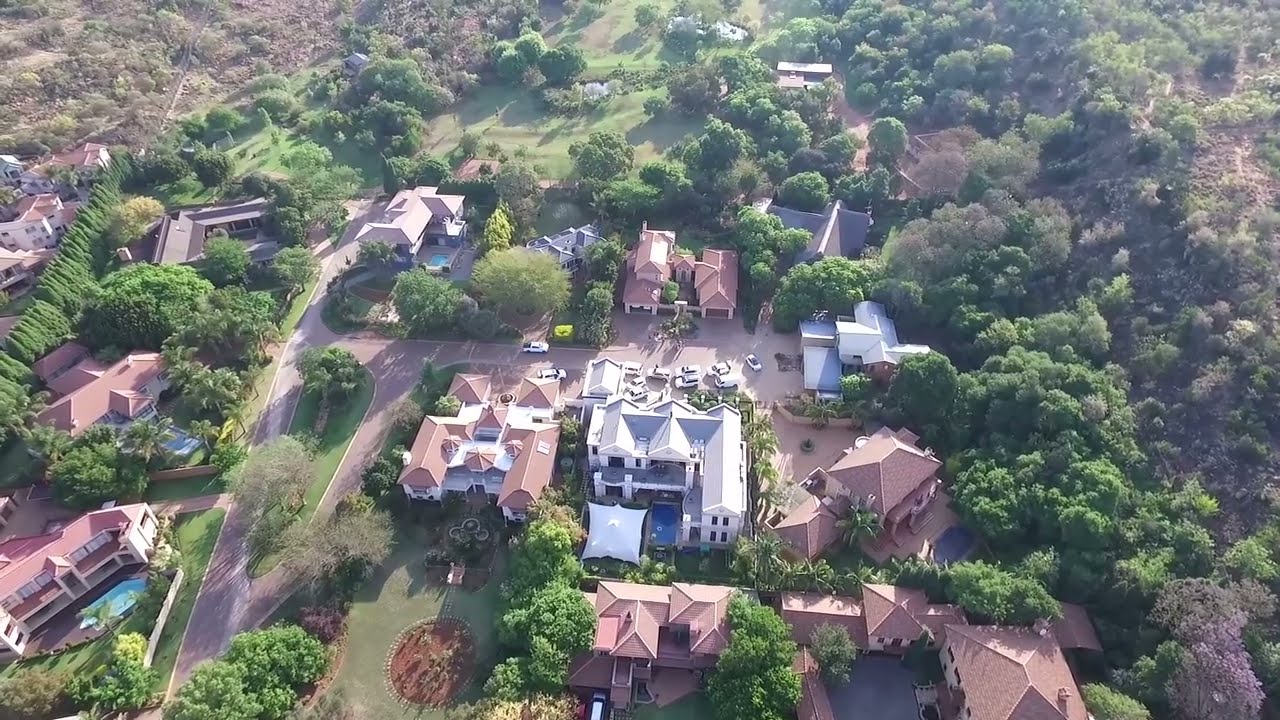The image provides an aerial view of a wealthy hillside neighborhood, featuring approximately 10 to 15 large homes, many resembling mansions. Most homes have roofs in varying shades of light brown and terracotta, except for one in the center with a gray roof, standing out as possibly a three-story structure. This central house is distinguished by a swimming pool in the backyard and multiple white vehicles parked in front. To its left, there's a new home under construction, followed by a column of three homes with two light brown roofs, one of which also has a swimming pool. The entire neighborhood is interspersed with landscaped gardens, palm trees, and other tall trees, providing an almost secluded atmosphere. Roads wind through the area, marking the separation between the houses. Towards the right side of the image, the trees and terrain become denser, transitioning into a large woodland area with dry land visible at the top corners. The top center of the image reveals a lush green area, possibly a golf course, further accentuating the luxurious nature of this estate.